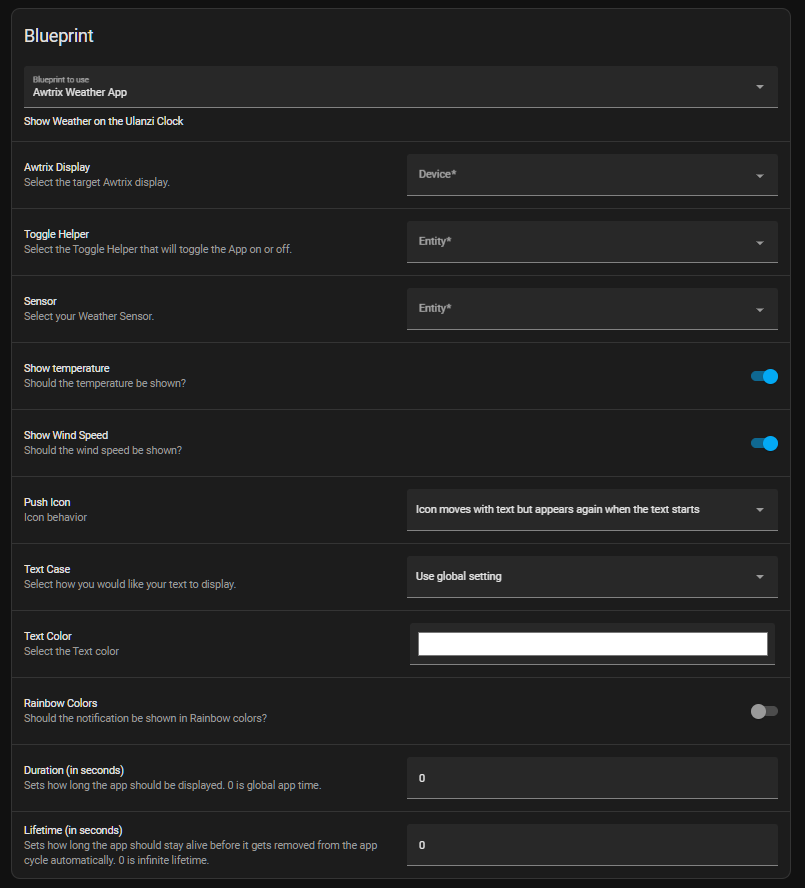This image depicts an electronic tablet displaying a sophisticated configuration interface for a weather application. The interface features a sleek black background with crisp white lettering. In the upper-left corner, there is a label titled "Blueprint," accompanied by a drop-down menu labeled "Autrix Weather App." Beneath this, another drop-down prompts the user to show weather data on an "Ulanzi Clock."

The interface includes several selectable options to customize the user experience further. Users can select the target display, labeled "Avatrix Display," via a drop-down menu. There are additional configurable elements, such as a drop-down for devices, a toggle for helper settings, and a current selection indicator for the entity, which is set to "sensor."

Additional settings include toggles to display temperature and wind speed, both of which are currently enabled. An "icon behavior" option allows the icon to move with the text but reappear when the text restarts. Text color customization is available, with the current selection set to white. A "rainbow colors" toggle for notifications is turned off.

Lastly, the interface shows fields for "Duration in seconds" and "Lifetime in seconds," both currently set to zero, indicating they have not been configured. The detailed, user-friendly layout suggests advanced customization capabilities for monitoring and displaying weather-related information.